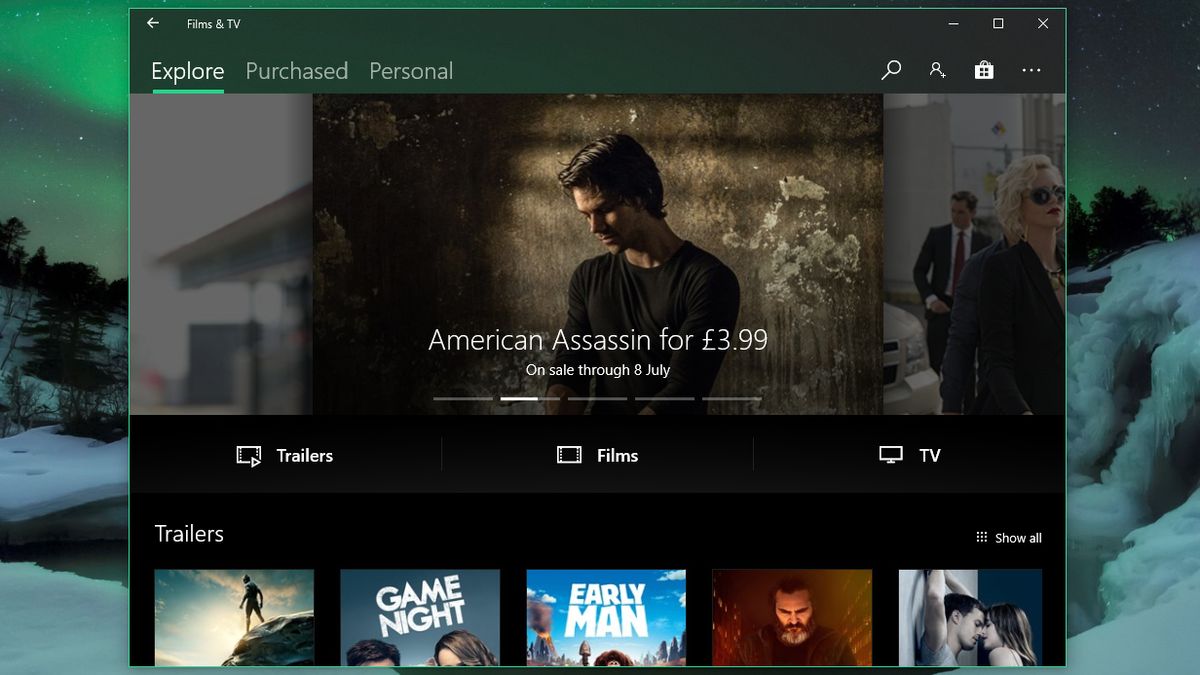The image depicts a computer screen with a website open, featuring a scenic screensaver in the background. The screensaver showcases a serene nighttime winter landscape, complete with a snow-covered ground, a body of water, and the mesmerizing Aurora Borealis illuminating the sky. In the foreground, there's a pop-up window labeled "Film and TV" with clickable tabs for "Explore," "Purchased," and "Personal." The central content of the window advertises the movie "American Assassin" on sale for $3.99, with an offer valid through July 8th. Below this advertisement, there are categories listed such as "Trailers," "Films," and "TV," with a specific focus on "Trailers" at the bottom of the pop-up. The trailer section displays five different movie thumbnails; however, only two titles are fully visible: "Game Night" and "Early Man," while the other three are partially obscured, rendering their titles unreadable.